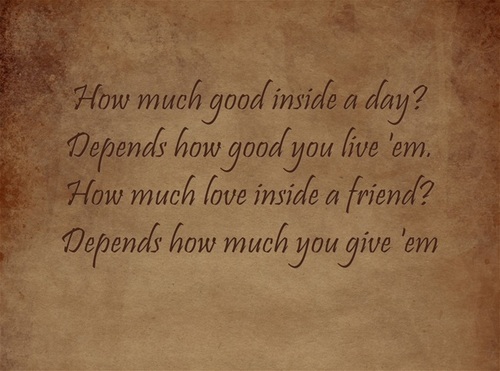The image features a background that mimics the appearance of aged, textured paper with a predominantly light brown center and patches of darker brown around the edges. Overlaying this background, there is a centered paragraph of text in a medium-sized, dark brown cursive font. The text reads: "How much good inside a day? Depends how good you live them. How much love inside a friend? Depends how much you give them." The overall aesthetic of the image, with its dark brown italicized lettering and vintage paper look, conveys a nostalgic and thoughtful message suitable for a social media or online quote.